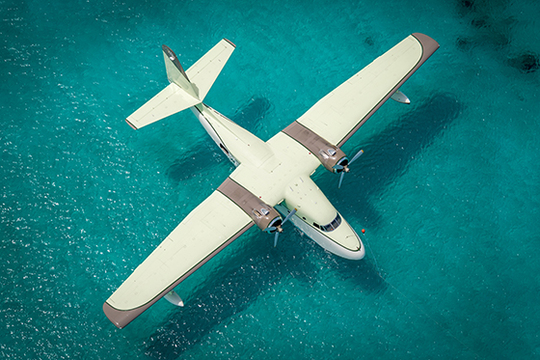The image is an aerial photograph capturing a small, white airplane with gray accents, flying low over a vibrant, clear blue body of water. The airplane, which could be a sea plane or a charter airplane, features two small propellers and minimal windows including the front pilot window and a couple at the back. The water beneath the plane is strikingly clear, revealing faint objects underneath and suggesting a tropical or island location. Both the airplane and some submerged objects cast shadows on the water, enhancing the clarity and detail of the scene. The well-lit photograph highlights the serene, picturesque quality of this potentially idyllic and hard-to-reach locale.